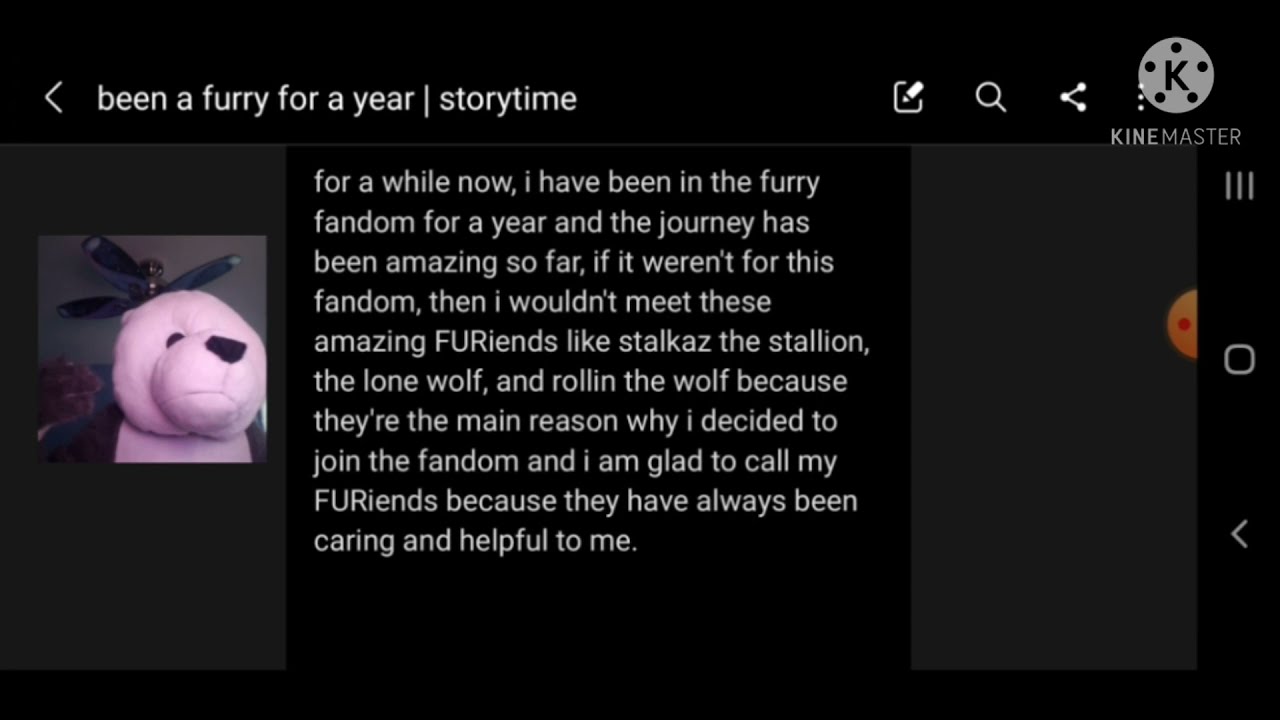The image is a screenshot, likely from the KineMaster app, of a website or app comment section. The background is completely black with a thin gray line at the top, containing the title in white font "Been a Furry for a Year Storytime" on the left, and app symbols on the right. Underneath the title, there's a small photograph on the left of a light pink teddy bear with a ceiling fan in the background. Next to this picture, there's a paragraph in white font against the black background, detailing a person's experiences in the furry fandom. The text reads: "For a while now, I have been in the furry fandom for a year, and the journey has been amazing so far. If it weren't for this fandom, I wouldn't have met these amazing fur friends like Stock the Stallion, the Lone Wolf, and Rollin the Wolf, because they are the main reason why I decided to join the fandom and I’m glad to call them my fur friends because they have always been caring and helpful to me." On the right side of the image, there are symbols, a gray block, an orange half-circle, and additional app icons resembling a home screen and navigational tabs, indicating it's a mobile screenshot.